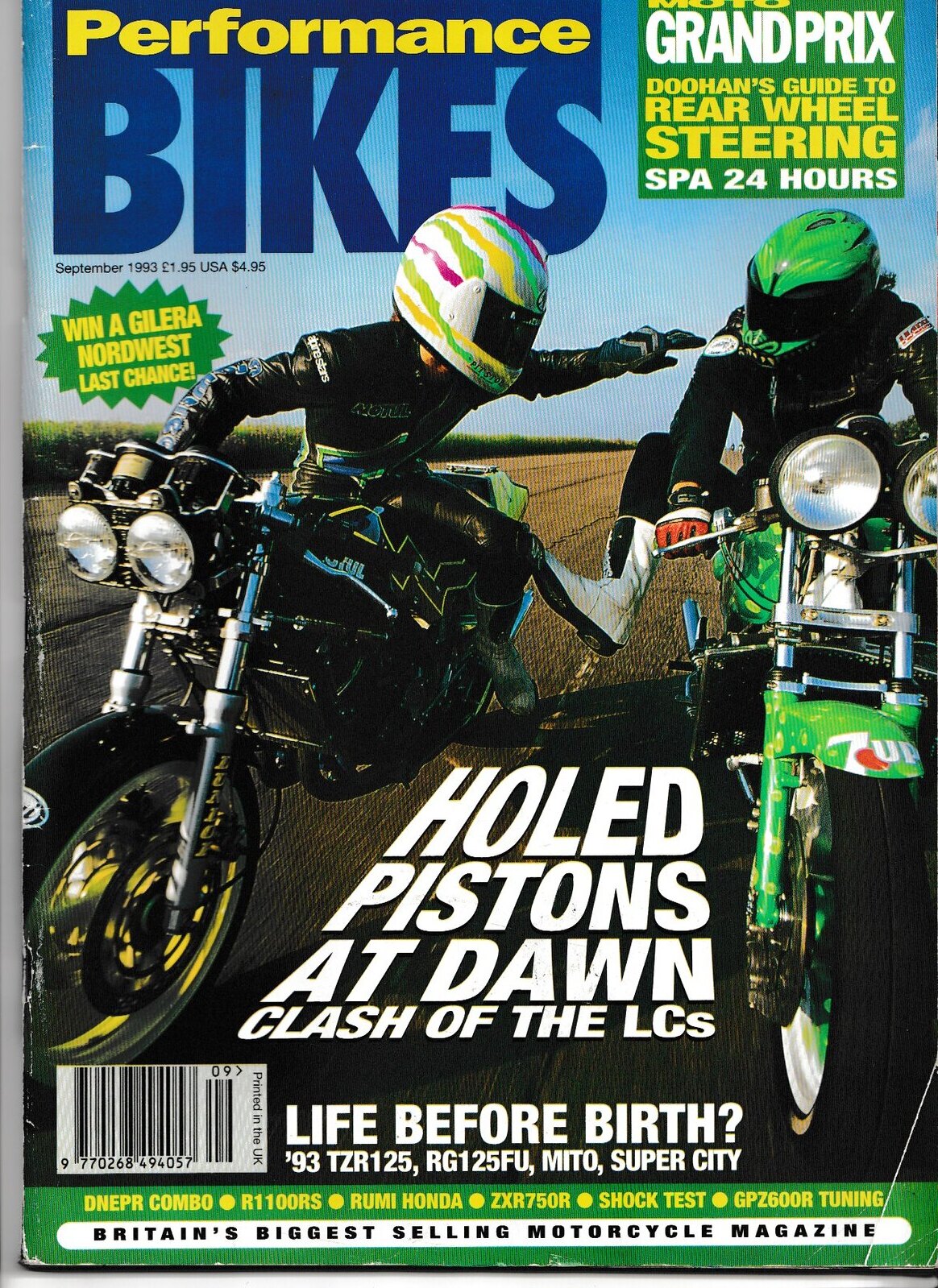This is the cover of the September 1993 issue of Performance Bikes magazine, marked at £1.95 or $4.95 US. The focal point is a dramatic scene of two motorcyclists riding down a road. On the left, a rider with a white helmet bearing green, yellow, and pink stripes reaches back toward the rider on the right, who is attempting to kick them. The latter rider's bike is painted green with "7Up" branding and they wear a matching green helmet; both riders are dressed in black motorcycle gear. The prominent headline between them reads "Hold Pistons at Dawn: Clash of the LCs" in white text. 

In the top left corner against a clear blue sky, in contrasting blue and yellow text, it reads "Performance Bikes." Below this, a green starburst highlights a yellow text promo: "Win a Galera Northwest. Last Chance." On the top right, another green box contains various headlines: "Moto Grand Prix, Doohan's Guide to Rear Wheel Steering, Spa 24 Hours." At the bottom section of the cover, additional text includes "Life Before Birth?" followed by "93 TZR125, RG125FU, Mito, Super City" and a green bar with yellow text listing: "DNEPR Combo, R1100RS, Roomie Honda, ZXR750QR, GPZ600R Tuning." The barcode is also located at the bottom. Finally, a standout white rectangle with black text proclaims: "Britain's Biggest Selling Motorcycle Magazine."